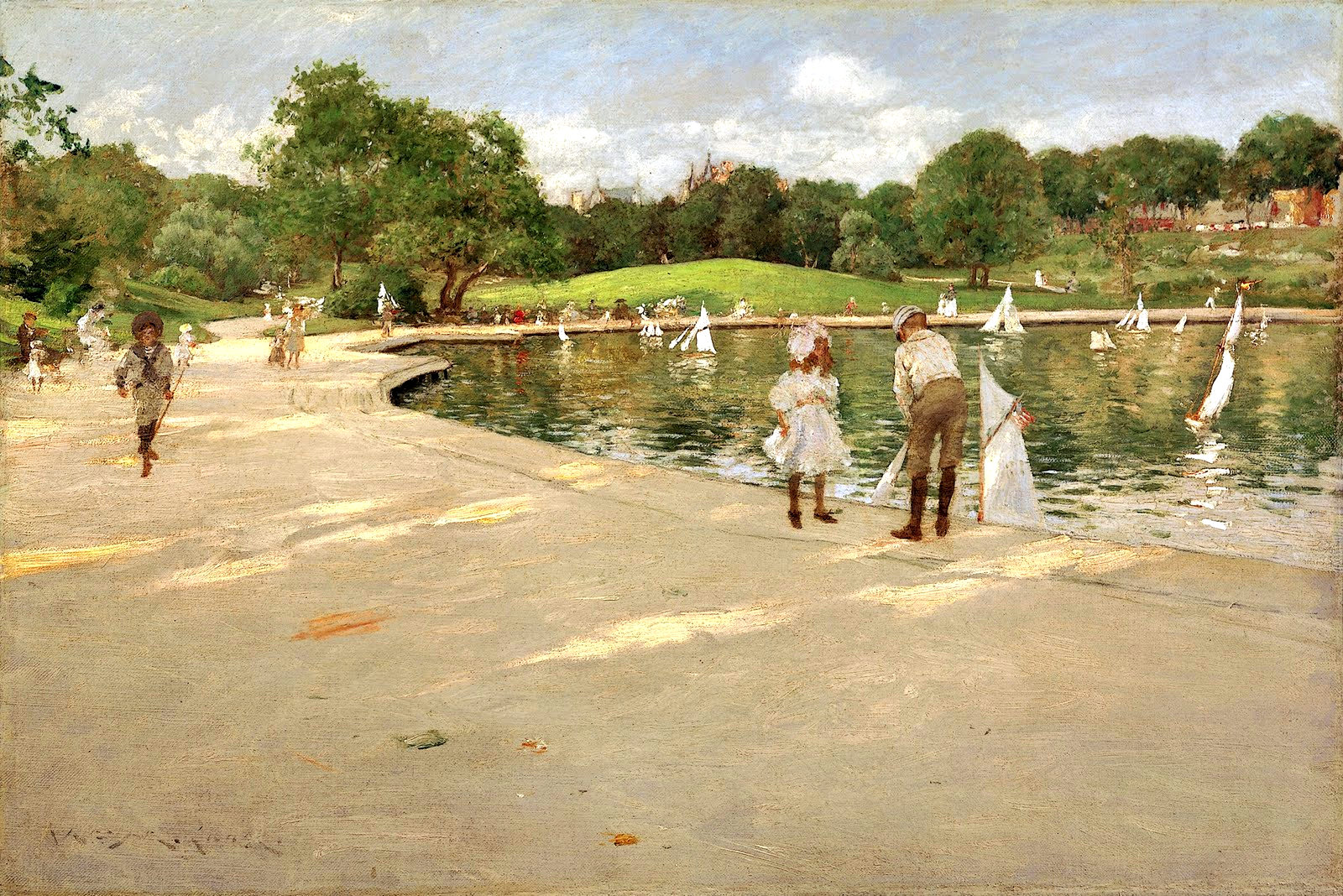The image is an oil painting depicting a scenic outdoor lake or pond during the daytime. The foreground features a concrete walking path that begins at the midline on the left-hand side and wraps around the lake, then continues horizontally across the image before disappearing off to the right. Along this path, several people are strolling about, enjoying the serene environment. On the right side of the painting, near the lake's edge, a man stands with his back to us, facing slightly left, and beside him a little girl facing him. Just to the right of center, a young boy dressed in brown breeches and a white long-sleeved shirt and cap stands with a young girl in a frilly white dress and cap, seemingly placing a toy sailboat into the water. The lake itself is reflective with numerous small sailboats floating on its greenish-gray surface. Beyond the lake, the landscape transitions into gently rolling grassy hills dotted with many trees. The sky overhead is cloudy, with gray clouds partially obscuring the blue. The entire scene exudes a peaceful charm, with the interaction between the figures and their surroundings creating a warm, inviting atmosphere.